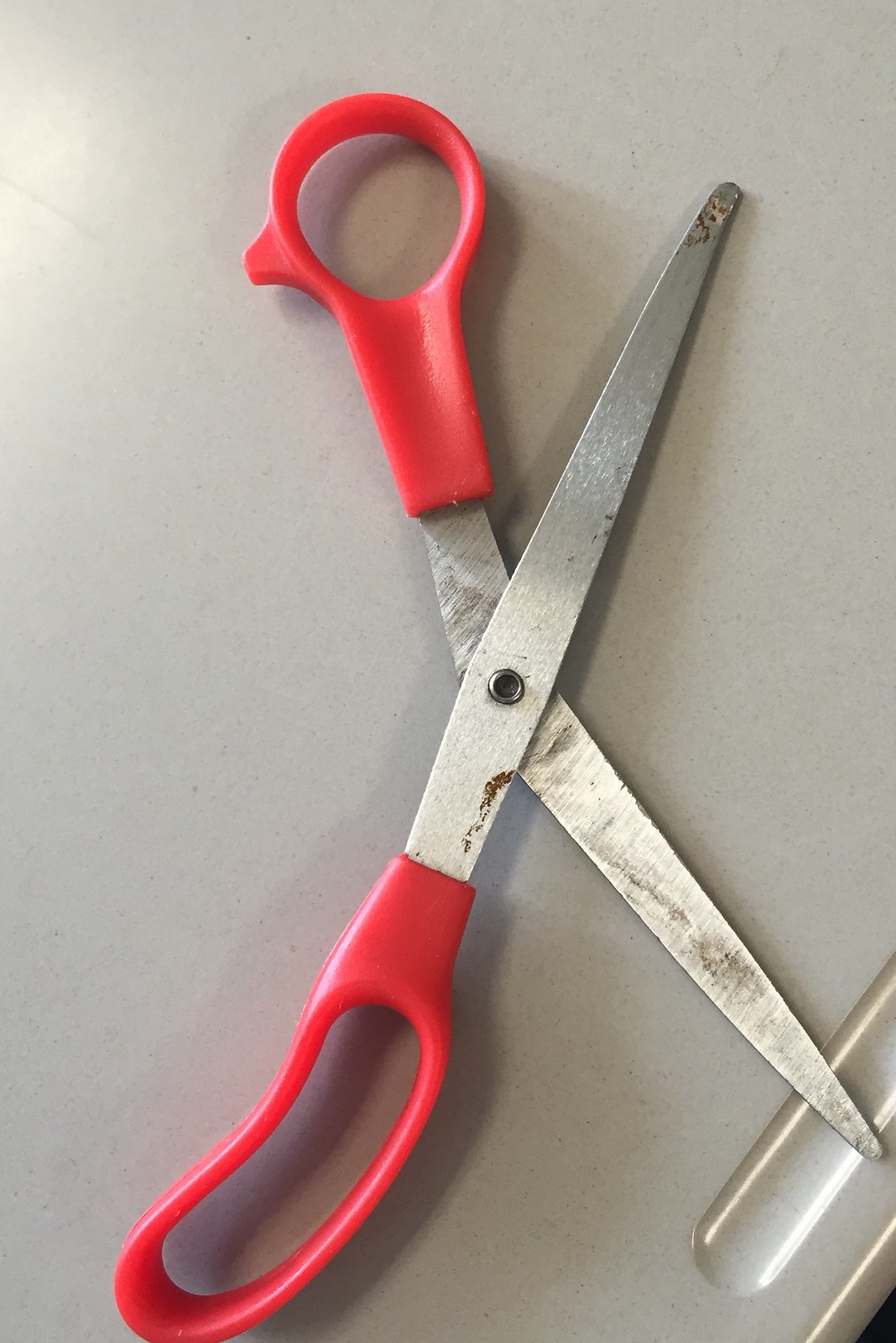This vertical image is a detailed close-up of a well-used pair of scissors with red plastic handles and a silver rivet or hinge in the middle. The blades of the scissors, which are metallic and noticeably stained with brown rust marks, are spread wide open. The handles, one wide for multiple fingers and the other narrower, likely for the thumb and with a small hooked extension, appear dirty and slightly worn. The scissors rest on a white or off-white table, which casts a shadow underneath the blades. There are indications of heavy use with scratches and dark residue on the blades. In the bottom right corner of the table, there is a small indentation shaped like a pill, adding a unique detail to the setting.